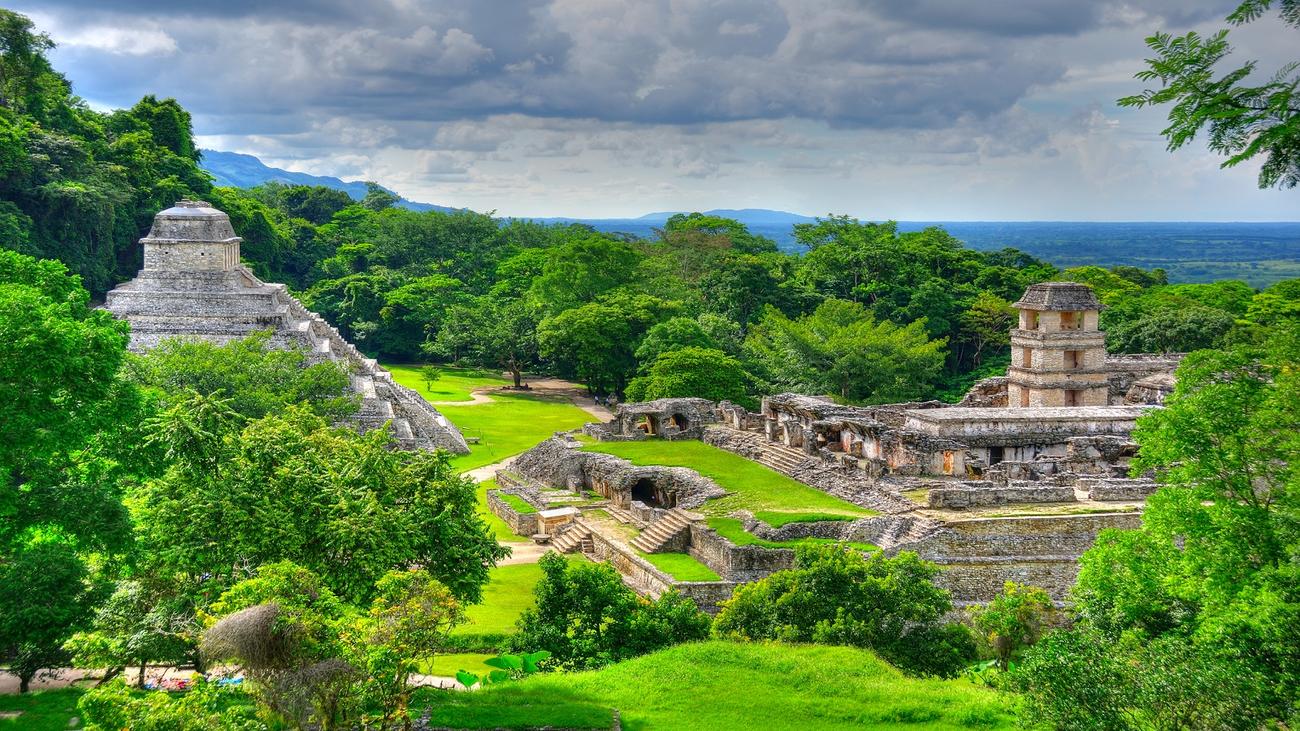This aerial photograph captures an expansive view of what appears to be Mayan ruins nestled in a lush, vibrant green landscape, possibly located in Mexico. The ruins are framed by dense foliage, with numerous brightly green trees and grass providing a stark contrast to the ancient, dark grey, and tan stone structures. Dominating the left side of the image is the tallest building, a towering structure partially obscured by trees. To the right, a sprawling, multi-layered ruin features two long, exposed layers topped with patches of grass. Showcased prominently in the middle is a significant pyramid-shaped building, possibly a ceremonial structure, characterized by its imposing height and an array of stairs leading upwards. The scene is completed by a backdrop of blue-tinged mountains and a cloudy sky laden with grey rain clouds, setting a dramatic tone as if a storm is approaching. This image vividly captures the timeless essence and grandeur of ancient civilizations amidst nature’s lush embrace.